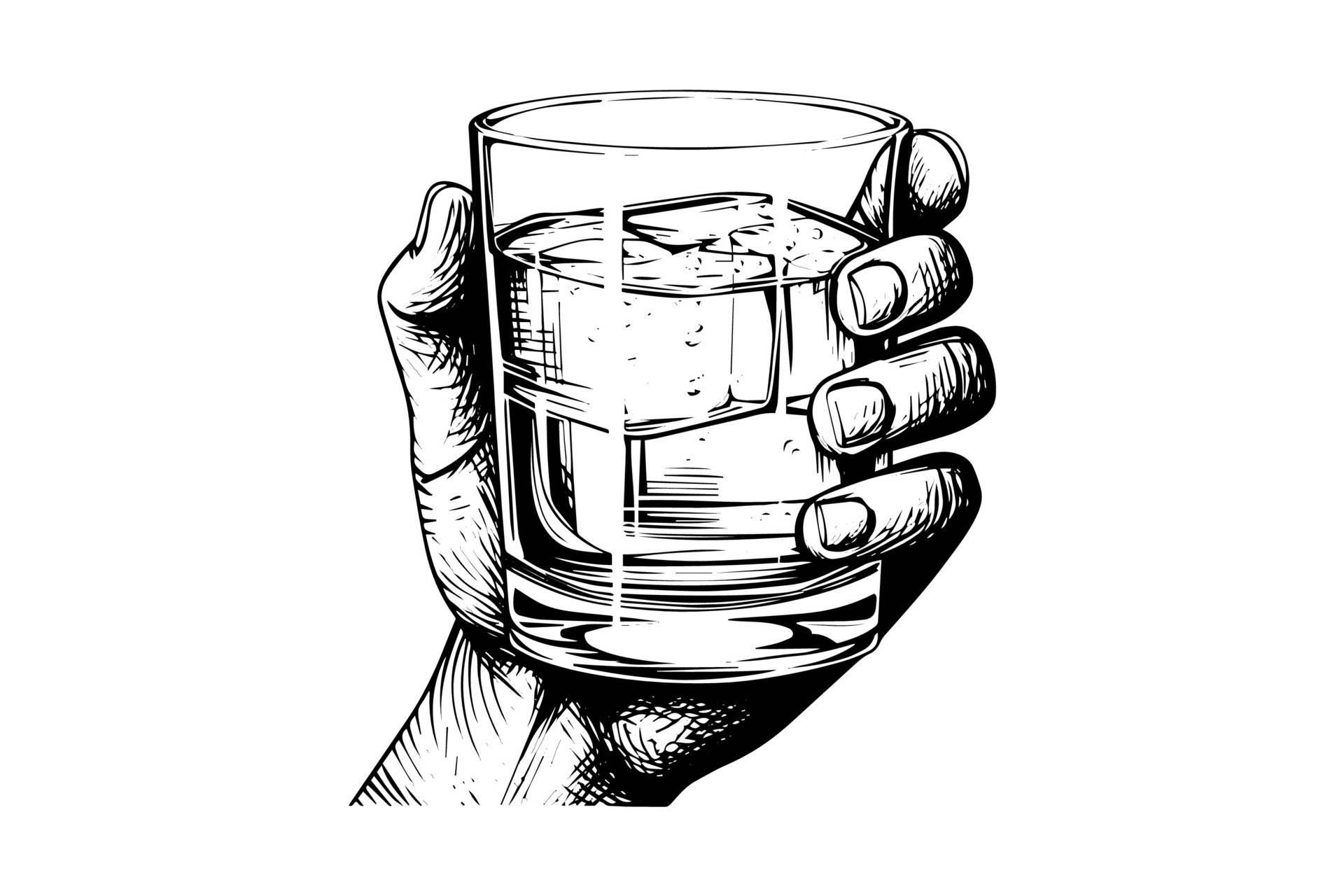A detailed black and white drawing showcases a left hand emerging from the bottom left corner, gripping a whiskey glass filled with a clear liquid and ice cubes. Rendered exclusively in thick black lines, the intricate details are depicted through fine strokes of the pen. The hand appears strong, with closely trimmed fingernails, and the thumb is positioned on the left side of the glass while the fingers grasp the right. The circular glass, which is about three to four inches tall and two to three inches wide, reaches just above the top finger. The drawing, characterized by its absence of color and background, relies solely on the interplay of black lines against a white canvas to create an evocative and detailed illustration.